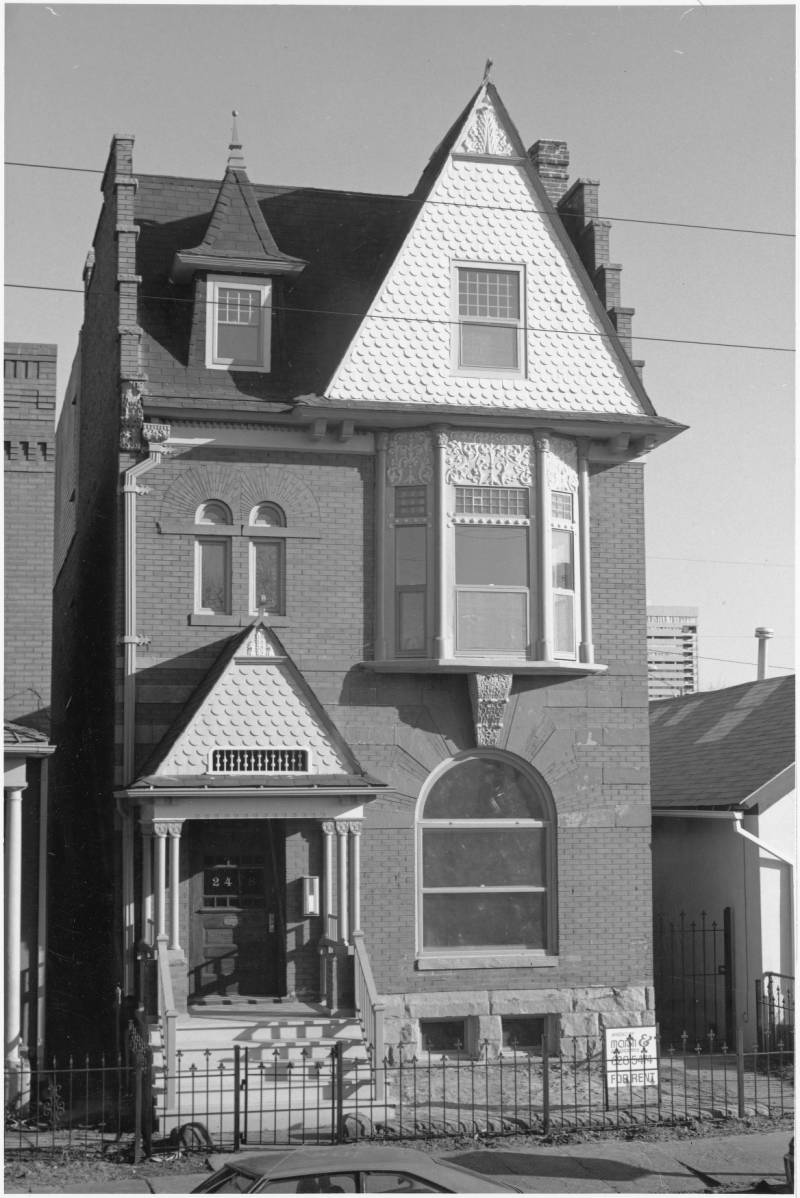The black and white photograph captures a traditional, stone-built, multi-level house from the 1960s or possibly the 1970s. The house is strikingly slender and vertical, featuring a distinctively pointy, white triangular roof on the top level. A smaller, matching triangular roof serves as an overhang above the front door. This three-story home has a simple layout: the first floor features one large window, the second floor has two sets of windows, while the top level also showcases two windows. The windows vary in design, with some having arches and others rectangular frames. The house is set behind a black iron gate, with a small staircase leading up to the front entrance. To either side of the house, other buildings are visible, indicating that the property has a very limited small front yard. The partially visible hood of a 60s-era automobile further enhances the nostalgic feel of the image.